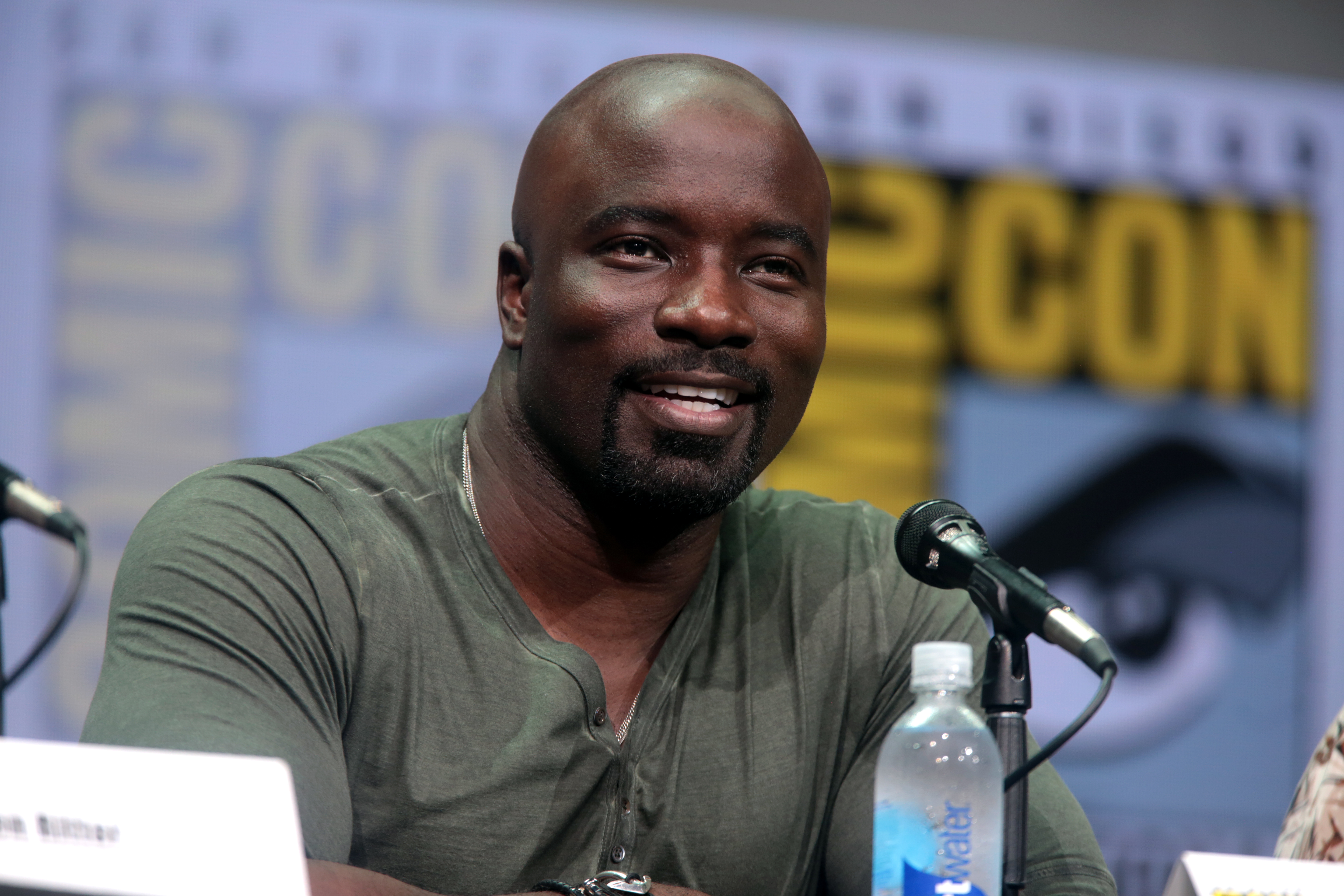A photograph captures a confident African American man, possibly in his early 30s, speaking into a black microphone at a Comic-Con event. The man, wearing a dark green t-shirt with an indistinguishable item hanging near its center, sports a goatee and a slight smile as he engages with the audience. In front of him on the desk is a bottle of Smartwater and several name cards, though the text on these cards is unclear. The backdrop features a blurred banner with discernible letters "C-O-N," indicating the event, but it's too blurry to read fully. The man exudes a cool and comfortable demeanor, suggesting he is well-versed and recognized, possibly hinting at familiarity as a public figure or athlete.